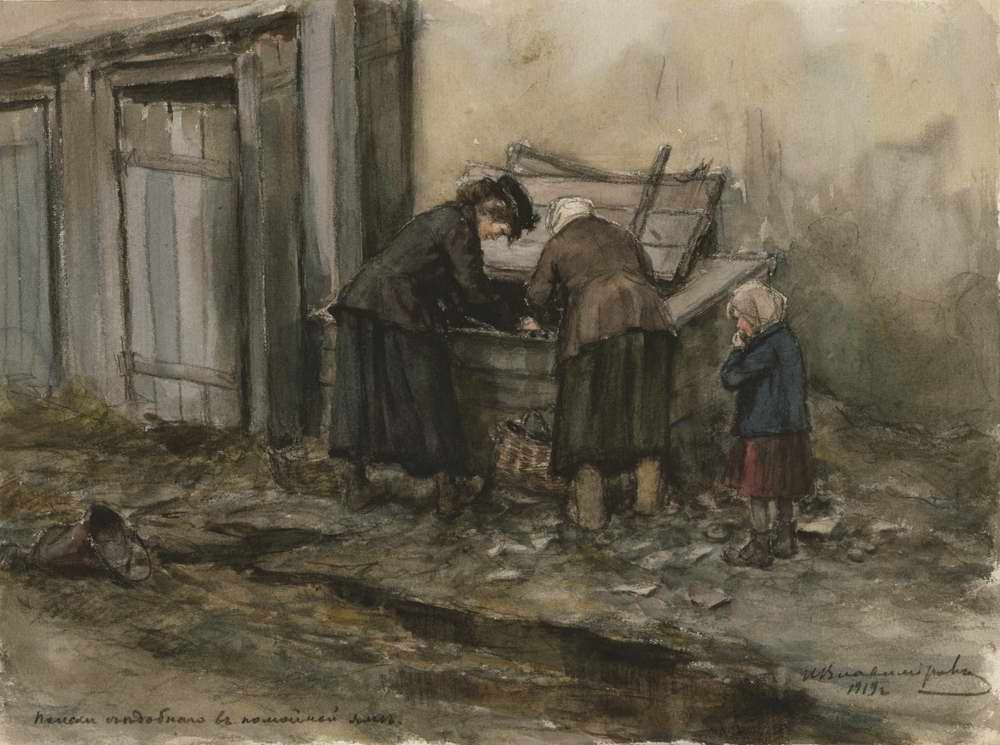This image is a detailed painting from 1919, depicting a grimy alleyway behind a dingy beige building with two dilapidated wooden doors on the left. The ground is littered with trash and murky water, emphasizing the cold and dirty ambiance. Central to the scene are three figures: two women and a small child. 

The woman on the left is clad in a black dress and a black hat, while the other woman, who appears older, wears a brown jacket over a black dress, brown boots, and a white bonnet. Both women are bent over, rummaging through a box or dumpster, their intent and precise actions suggesting they're scavenging for food.

Standing to their right is a small child, looking on with curiosity and a hint of sadness. She is dressed in a blue jacket, a red skirt, black boots, and a white scarf or bonnet, with her hand in her mouth.

The painting employs an old-school technique, capturing the essence of early 1900s attire and atmosphere. In the bottom right corner, there is an illegible signature followed by the year "1919." The scene is likely set during the day, bathed in diffuse light that enhances the overall mood of desolation and hardship.